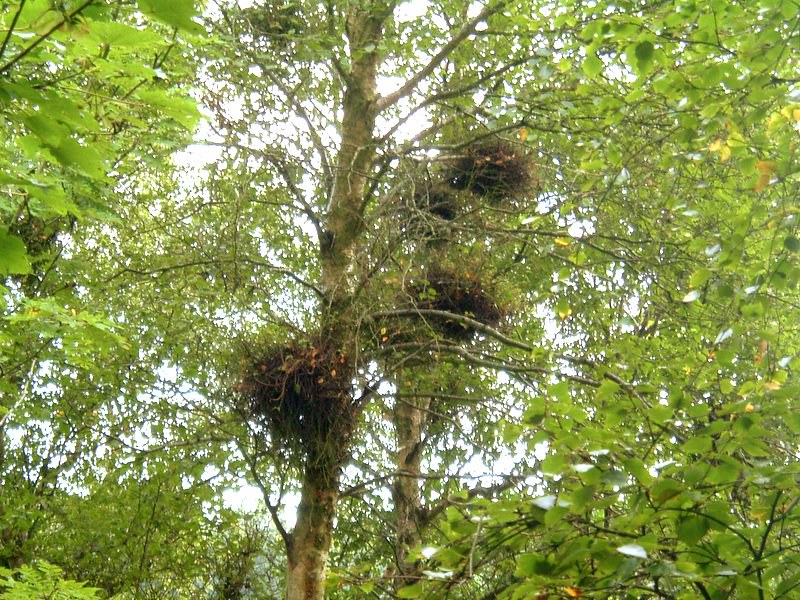This vibrant close-up photo captures the intricate details of several birds' nests nestled within the upper canopy of a tree, situated in a lush forest area. In the image, three well-defined nests made of dark brown sticks stand out, with possibly two more faintly visible in the background. The nests, almost round-shaped and appearing quite messy, are positioned on various branches extending from a prominent tree trunk. Surrounding the nests, the branches spread outwards, with light green leaves sprouting on the left and right sides, contributing to the rich greenery and dense foliage of the canopy. The background features patches of white light filtering through the leaves, suggesting a clear sky above, enhancing the natural serenity of the scene. This photograph distinctly showcases the quiet beauty and complexity of avian architecture in a pristine forest setting.